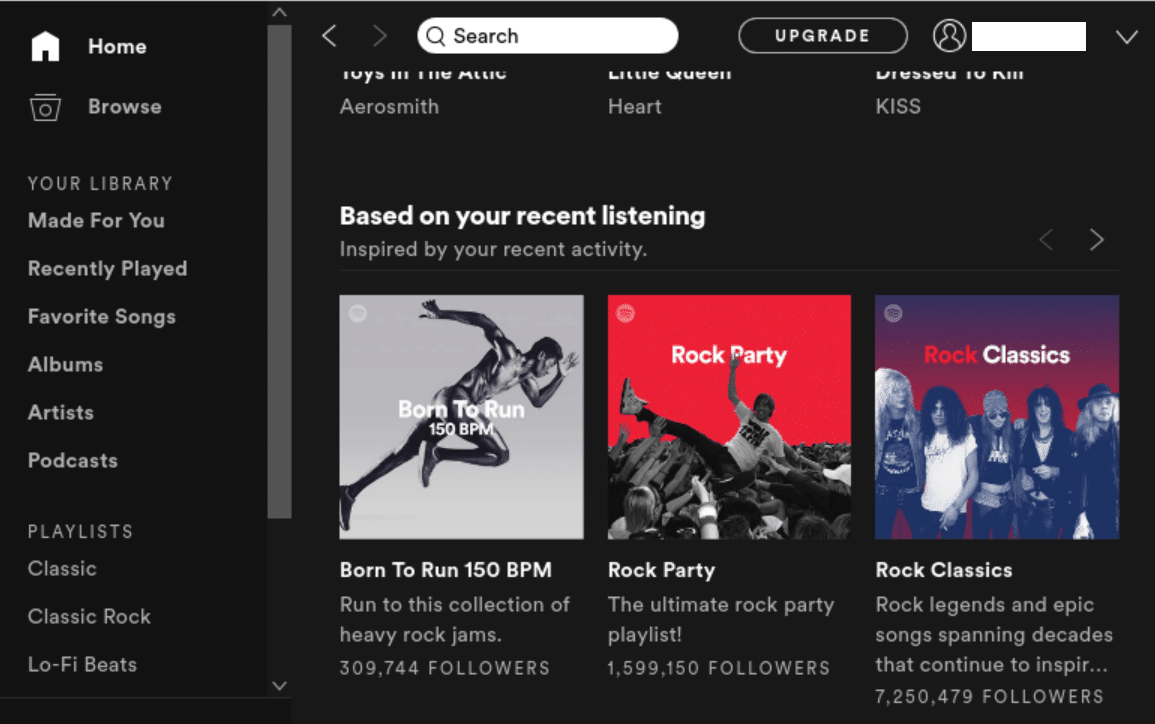In this image, we observe a detailed interface layout featuring various navigational and content elements. 

**Top Left:** A "Home" button is present with a tent logo beside it. Below "Home," there's a "Browse" option, followed by "Your Library." Under "Your Library," multiple categories are listed: "Made for You," "Recently Played," "Favorite Songs," "Albums," "Artists," "Podcast." Further down, under the "Playlist" section, there are specific playlists such as "Classic," "Classic Rock," and "Lofi Beats."

**Middle Right:** Adjacent to the categories, there is a vertical scroll bar with arrows pointing up and down on either end, separated by a large light gray rectangle in between.

**Top Right:** An arrow pointing down is visible, typically indicating a dropdown menu. To its left, a white rectangle obscures what is presumably the username. Further to the left, a prominent "Upgrade" button is displayed in a bubble. Additionally, there is a chat bar labeled "Chat."

**Bottom Middle:** Three prominent content squares are displayed: the left square is titled "Born to Run," the middle square "Rock Party," and the right one "Rock Classics."

The layout combines intuitive navigation with easily accessible music categories and playlists, making for a user-friendly experience.